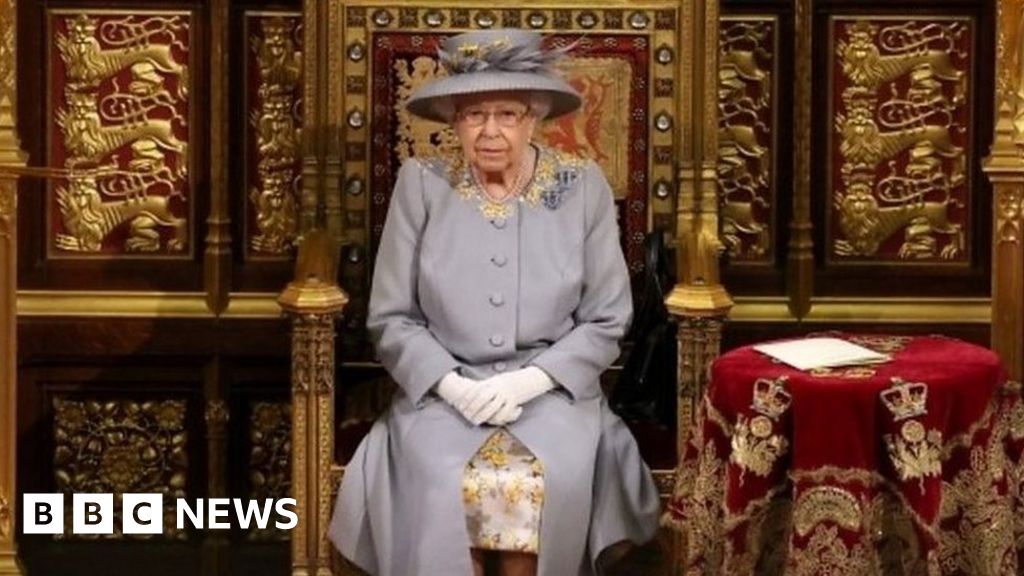This image is a screenshot featuring the former Queen of England, Queen Elizabeth, captured in a still photograph. Seated on a grand, dark gold throne adorned with intricate dark red velvet upholstery and circular designs, she exudes a regal presence. The throne is remarkably detailed, with golden arms and trim extending up the very tall rectangular back, which is embellished with shiny, diamond-like jewels. The dark red cushion includes what appears to be a red dragon design. Surrounding the throne is a wall with lavish dark gold and red designs that include lion-like creatures with crowns and golden floral trims.

The Queen herself is wearing a meticulously coordinated outfit: a light gray coat with matching gray hat decorated with gray feathers at the front. Her coat, buttoned down the center, features an elegant collar adorned with small yellow flowers, displaying a hint of a white dress beneath, which also has tiny yellow flowers. She completes her attire with white gloves, her hands resting gracefully one over the other in her lap, and glasses perched on her face. Notably, the light blue hat and coat mentioned by one of the reviewers seem to be a misinterpretation, as the detailed descriptions align more consistently with the light gray attire adorned with yellow floral accents. The bottom left corner of the image features the "BBC News" label, indicating its source and the context of the report.